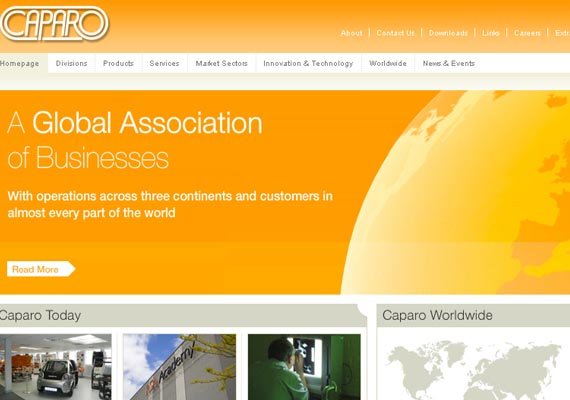The webpage screenshot features the title "Capero" prominently displayed at the top against an orange background with crisp white text. The navigation bar is replete with various sections including About, Contact Us, Downloads, Links, and Careers. Multiple tabs are visible, labeled as Homepage, Divisions, Products, Services, Market Sectors, Innovation and Technology, Worldwide, and News and Events.

Dominating the center of the page, there is a prominent section with an orange background featuring a sun-colored graphic. It boasts the text: "A global association of businesses with operations across three continents and customers in almost every part of the world." Beneath this text, a "Read More" button provides further information. 

The "Capero Today" section showcases a diverse array of images. One image depicts a sleek gray and black car, another shows the exterior of a building labeled "Academy," and a third captures a person examining an x-ray through specialized equipment, suggestive of a healthcare context.

Further down, the "Capero Worldwide" section features a detailed world map in gray set against a white background, emphasizing Capero's global presence.